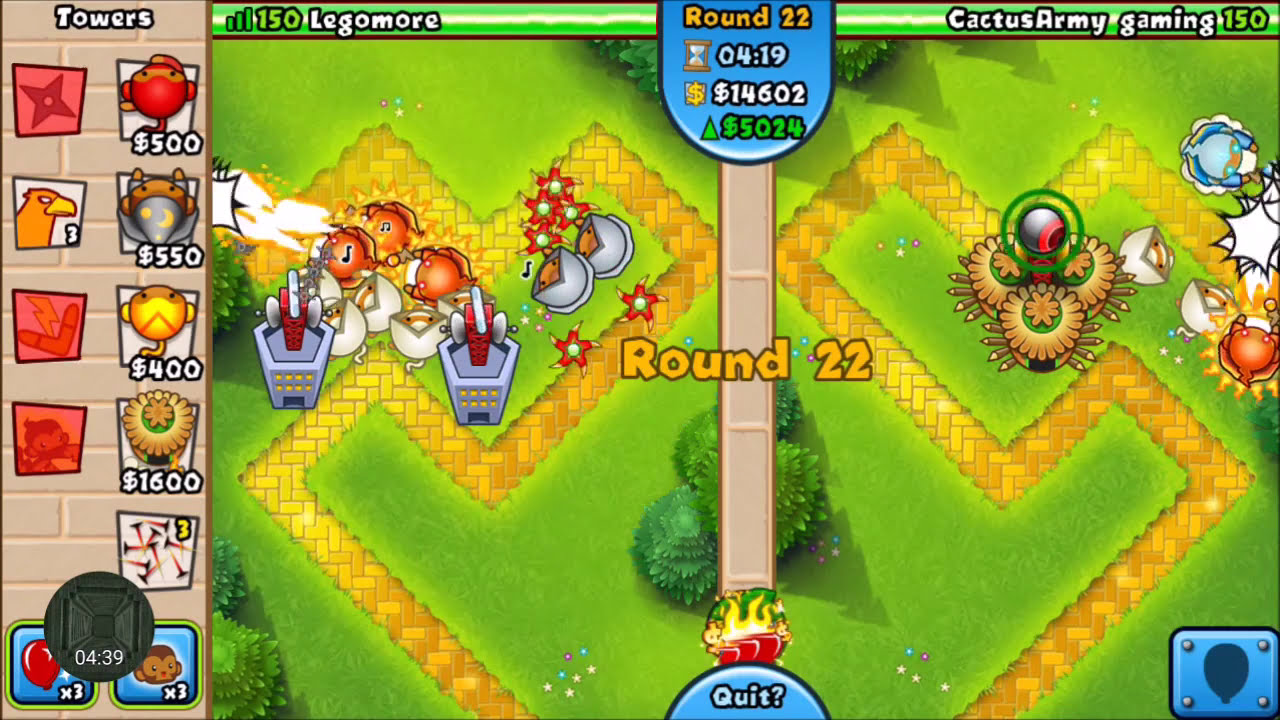The image depicts a screenshot of a mobile tower defense game set on a maze-like, yellow-brick pathway in a grassy field. The game is at round 22, highlighting a one-on-one competition between two players, Lego More and Cactus Army Gaming. The pathways include multiple turns and bends, lined with various defensive towers on both sides. The left side features city buildings with red towers and satellite dishes, while the right side showcases huts made of sticks with flower roofs. Several explosions are visible near the towers, indicating ongoing combat. The left panel of the screen lists purchasable towers and their prices, including $500, $550, $400, and $1,600, alongside images of shurikens and other defensive items. A time clock is positioned at the bottom left.